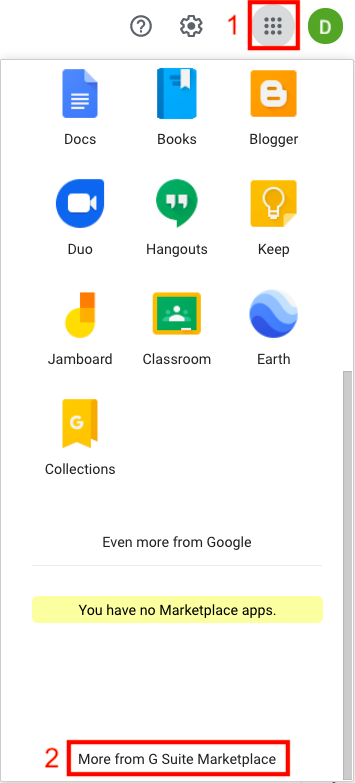This screenshot depicts a mobile device screen with various icons and elements. At the very top, the status bar displays several icons: a circle with a question mark inside, a grey gear icon, a red notification with the number '1', a grey circle containing 9 dots arranged in a 3x3 grid (possibly representing a menu or app drawer), all enclosed within a red square, and a green circle with the letter 'D' inside.

Below the status bar, the screen shows a collection of application icons predominantly related to Google services. These include:

- **Books**: Represented by a blue book icon labeled "Books."
- **Blogger**: Displayed with the Blogger logo.
- **Google Duo**: Depicted as a blue circle with a white camcorder icon.
- **Hangouts**: Represented by the Hangouts icon.
- **Keep**: Displayed with the Google Keep icon.
- **Jamboard**: Shown with the corresponding Jamboard icon.
- **Classroom**: Featuring a chalkboard icon.
- **Earth**: Represented by a wavy blue circle icon.
- **Collections**: Displayed with the Collections icon.

Towards the bottom half of the screen, there's a section labeled "More from Google," followed by black text on a yellow strip stating "You have no marketplace apps." Beneath this, another section reads "More from G Suite Marketplace," encased within a red rectangle, with a red notification showing the number '2' to its left.